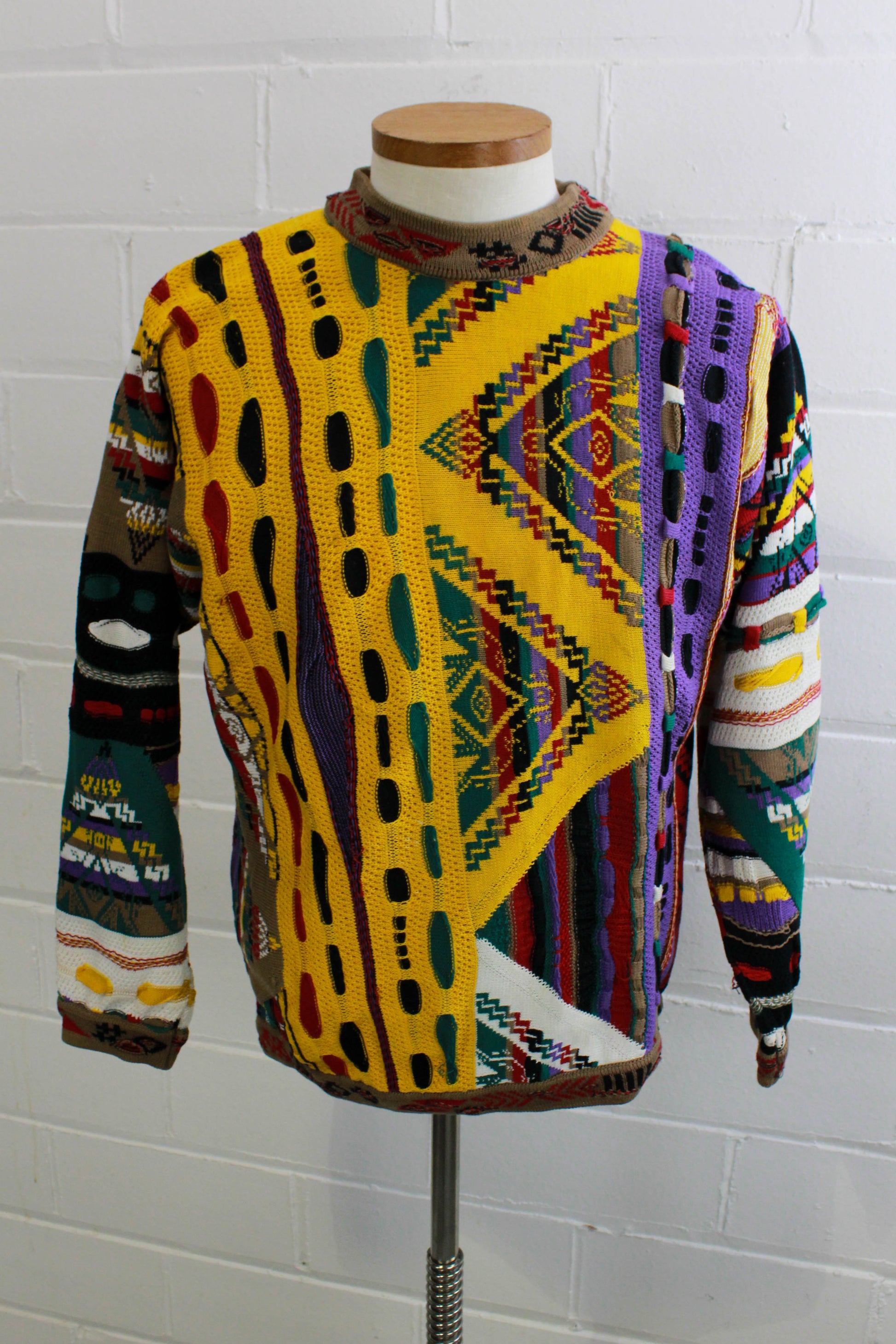The photograph showcases a vibrant, detailed sweater displayed on a mannequin against a white, slightly grayish cinder block wall. This men's sweater features a dynamic and colorful design, drawing inspiration from traditional African patterns. Dominated by shades of yellow, the garment also incorporates purple, red, black, green, brown, and touches of white. The front of the sweater is divided into three vertical sections: two primarily gold with zigzag and abstract patterns, and one with a prominent purple stripe. The right side has extra pieces of yarn sewn at the top, adding texture to the heavy, thick cotton knit. The sleeves are adorned with a multitude of geometric shapes, circles, squares, lines, and diagonals, making the sweater strikingly stylish and visually engaging.